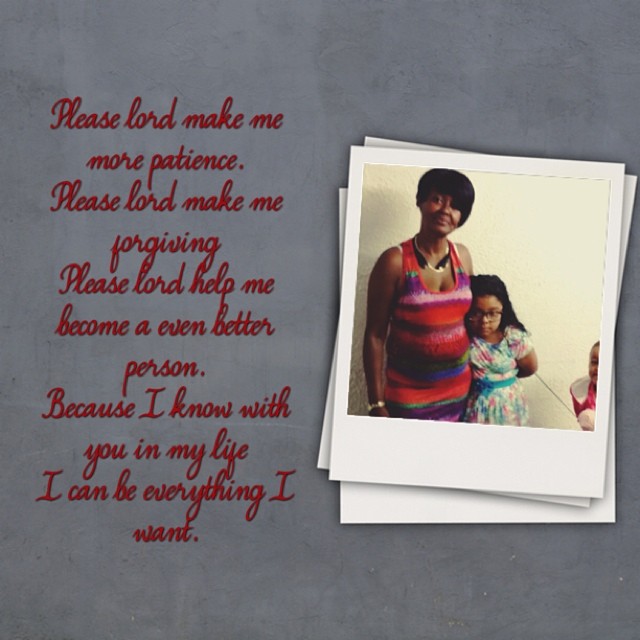The image features a gray, cement-like background. On the right side, several Polaroid photos appear scattered and slightly overlapping. The top photo prominently displays an African-American woman and a young girl. The woman, smiling, wears a multicolored striped dress with shades of red, purple, pink, and some blue and yellow. She has a short hairstyle. The young girl beside her, who appears to be hiding slightly behind the woman, wears glasses, has long dark hair, and dons a light dress adorned with pink and teal flowers. The girl has her arms folded behind her back. To the left of these photographs, red cursive text reads: "Please Lord, make me more patient. Please Lord, make me forgiving. Please Lord, help me become an even better person. Because I know with you in my life, I can be everything I want." This motivational message adds a heartfelt dimension to the image, making it suitable for social media or personal dedication.